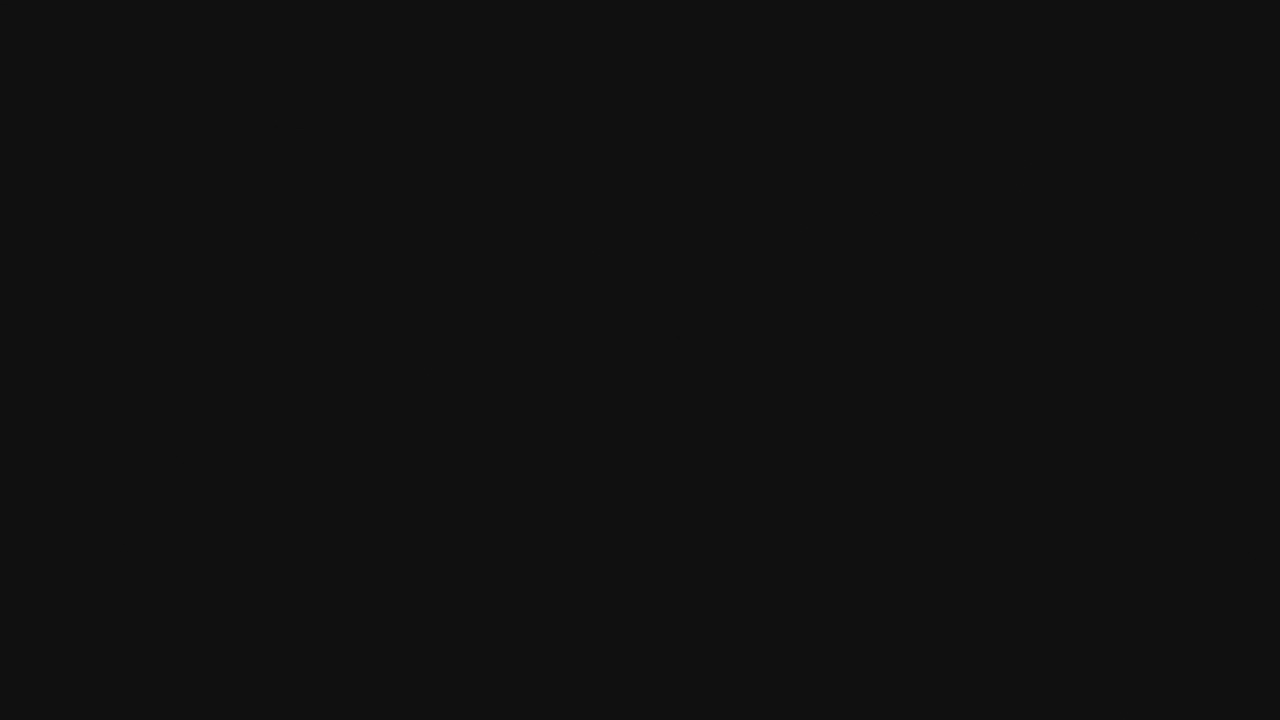The image displayed on the website is entirely black, devoid of any text, visual elements, or explanatory content. The horizontal image spans wider across the top and bottom than it does vertically along the sides. The blackness is deep and unbroken, showing no variations in shade or texture and free from any detectable interruptions. It encapsulates complete darkness without any evident reflections or light sources. Viewing from different angles—be it from the side, top, or bottom—yields no additional information or features. The dimensions closely resemble those of a standard website layout in width, though it may be slightly shorter in height. The uniform darkness and lack of detail suggest that, if this is content intended for a website, it might be erroneous or incomplete.